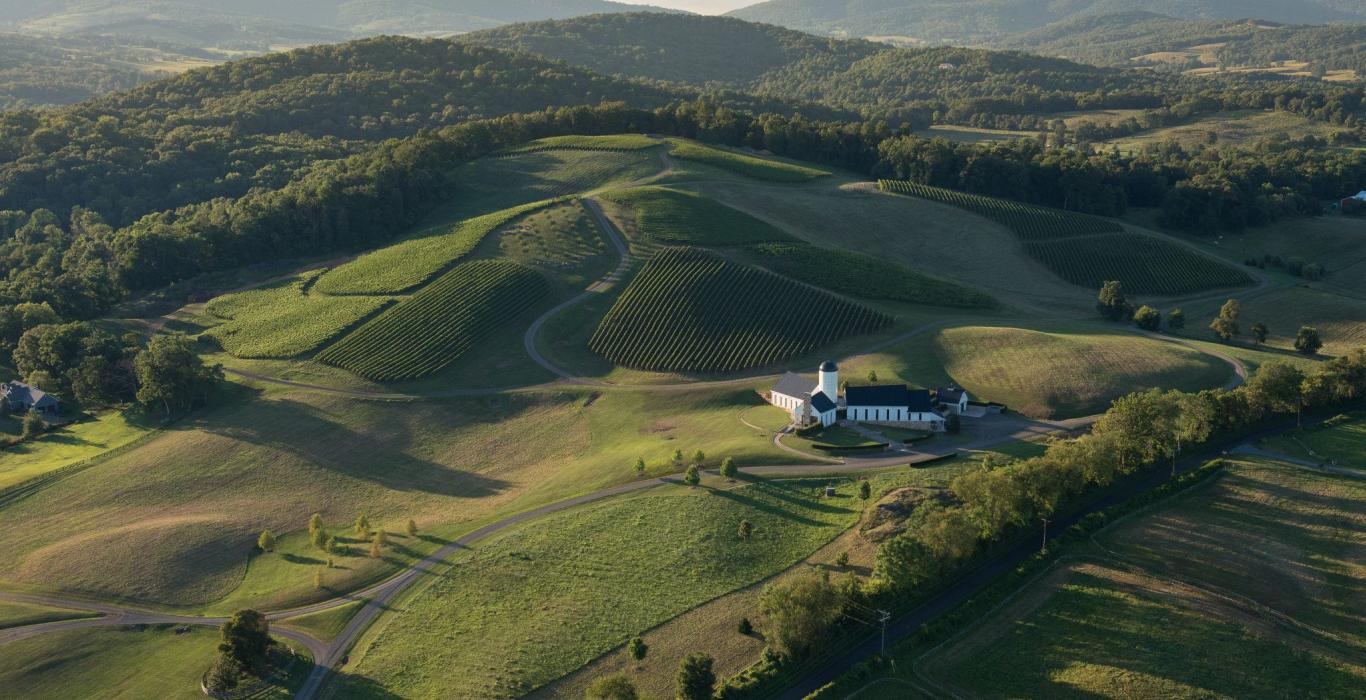This color aerial photograph, captured in landscape orientation during a bright day, showcases a vast expanse of hilly terrain interspersed with pastures and fields of green grass. Dominating the foreground is a white building with a dark-colored roof and a tower structure on its left side, which could be a farmhouse or a church. Surrounding the building is a sloping lawn of green grass, bordered by rolling hills and rows of crops. The hills in the background are densely covered with dark green trees, while several layers of mountains recede toward the horizon, adding depth to the expansive, rural landscape. Hay bales dot some of the fields, further emphasizing the agricultural nature of the area.